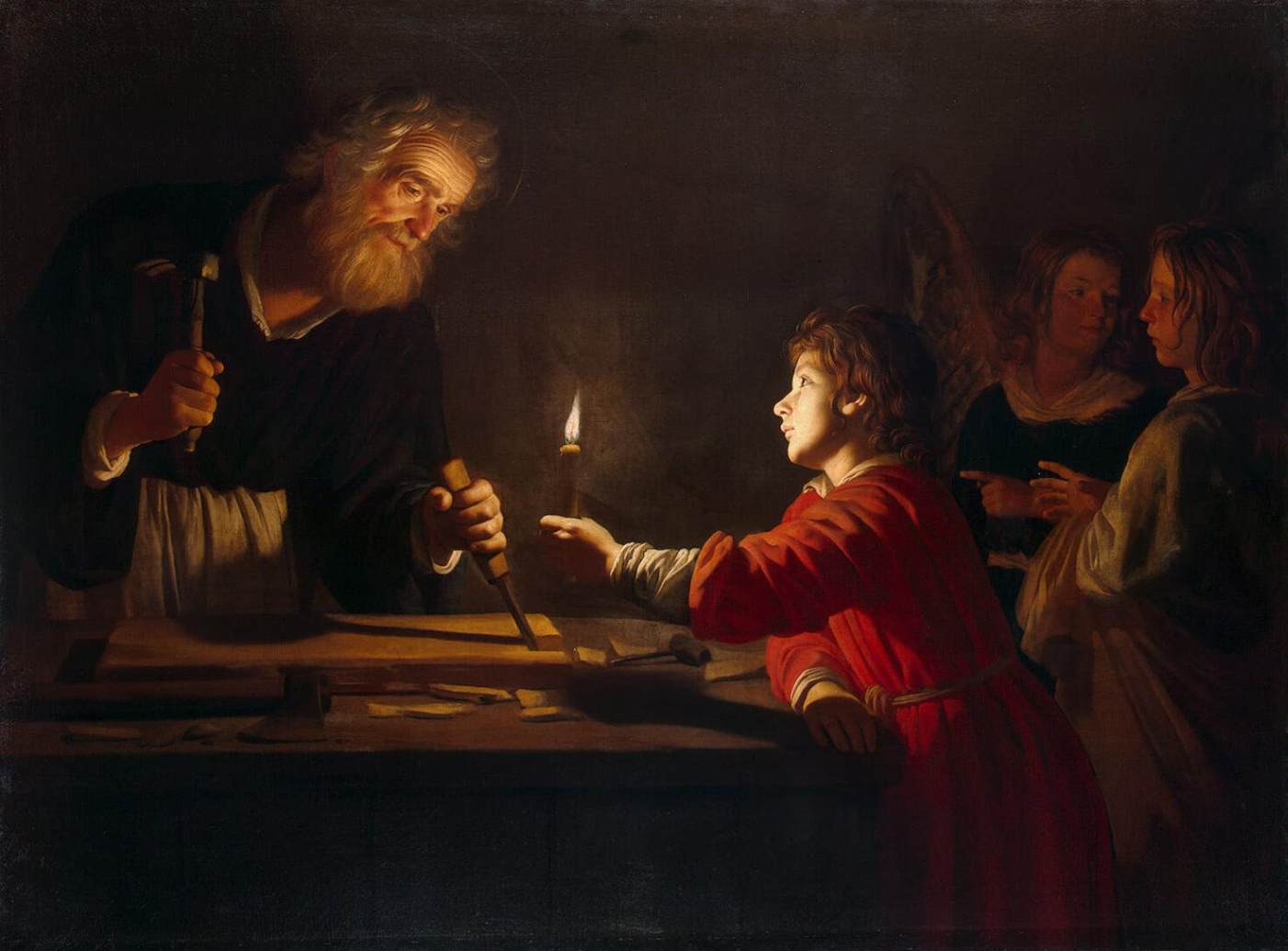This detailed painting, seemingly from the 18th or 19th century, depicts a dimly lit indoor scene with a group of people engaged in various activities. On the far left, an older bearded man, likely in his 50s or 60s, is deeply absorbed in his work, holding a chisel and hammer and possibly crafting something atop a table cluttered with woodworking tools and pieces of wood. He is dressed in a black robe with a dark white apron and seems focused on his task, illuminated by a candle held by a child next to him. The child, wearing a red robe, stands near the table, holding the candle to provide light for the older man’s work. To the right of the scene, two females, possibly the child’s mother and sister, are engaged in conversation, seemingly detached from the main activity. The females are dressed in contrasting robes, one in dark and the other in light colors. The overall palette of the painting includes shades of brown, red, black, gray, yellow, and tan, enhancing the darkness of the room except for the soft glow from the candle, highlighting the intimate and historical aura of the setting.